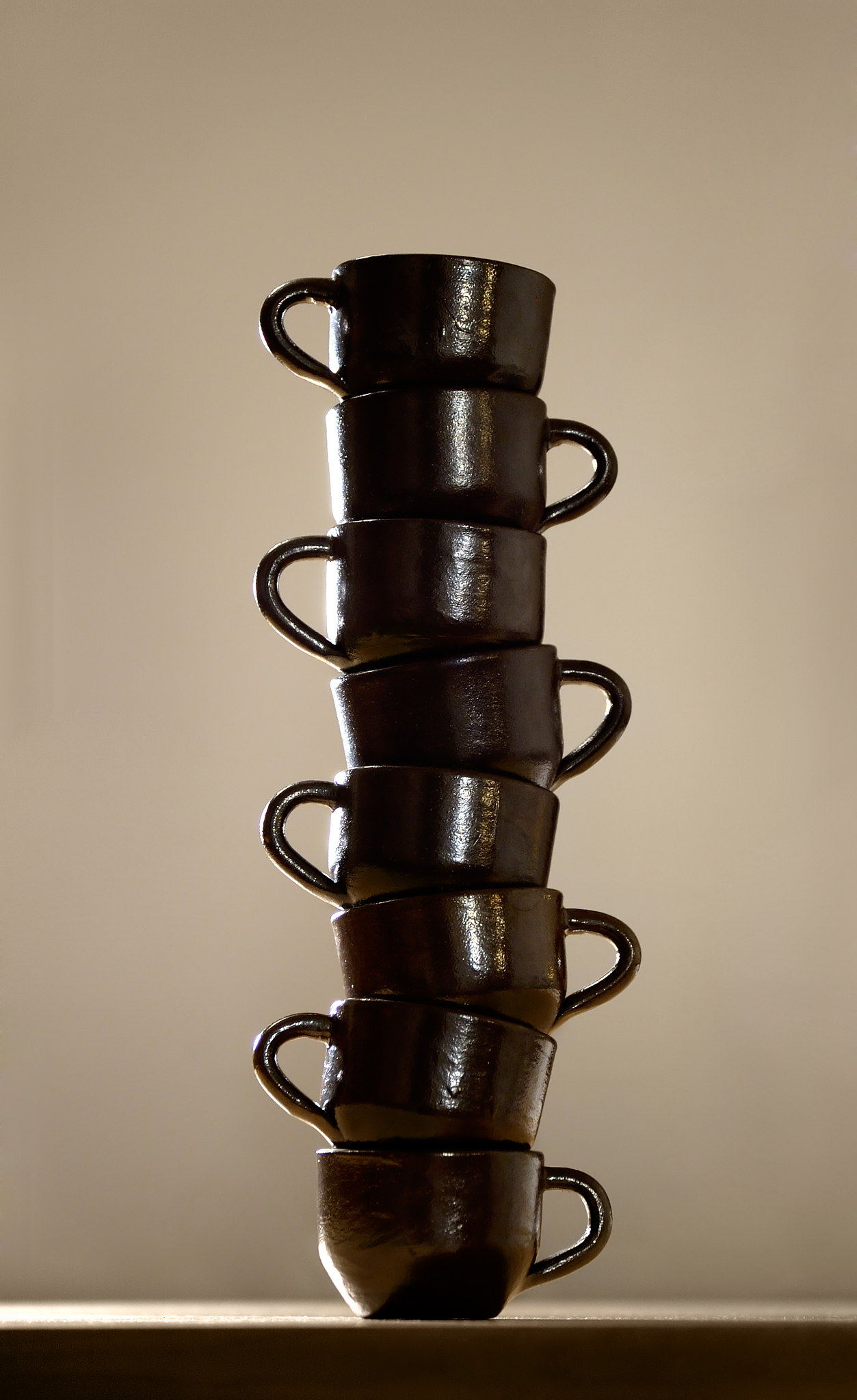The image is a detailed photograph of eight dark brown, coffee-colored ceramic mugs stacked on top of each other in a tower-like structure. The mugs alternate the direction of their handles: the bottom mug's handle faces right, the next left, and so on, creating a zigzag pattern. The mugs are stacked on a dark brown, wooden table situated at the very bottom of the photo. Light from the left side of the image illuminates the mugs, casting subtle reflections on their surfaces. The background is a plain beige or tan off-white wall, enhancing the simplicity and focus of the scene.